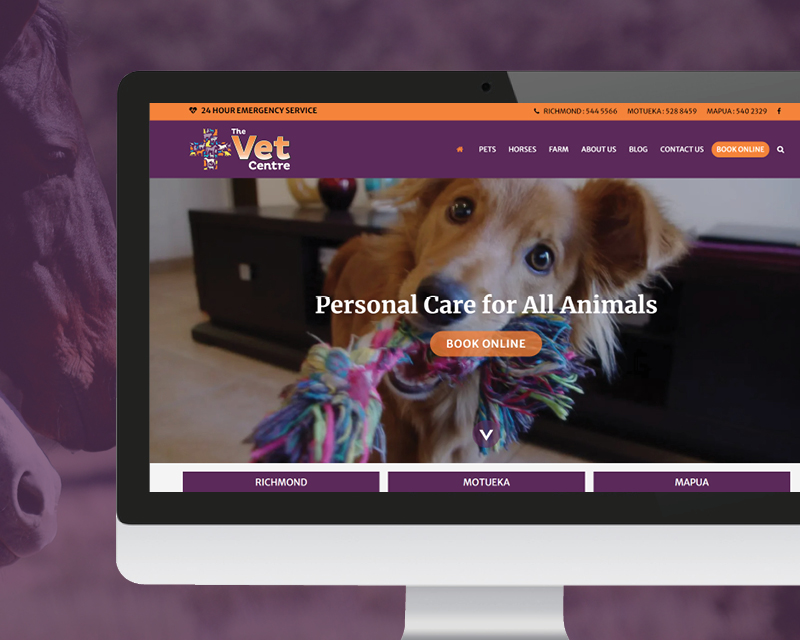This is a detailed screenshot from the VET Centre website, characterized by a vibrant palette of purple and orange. The topmost orange banner prominently features a small icon in the left corner indicating "24 Hour Emergency Service". Centrally placed in the banner is an old-school telephone handset icon accompanying various contact details in purple text: "Richmond 544-5566," followed by "Montuca 528-8459," and "Mapua 5402329." Just after these, a blue "F" of the Facebook logo makes its appearance.

Below, a purple banner displays the VET Centre logo alongside navigation options: "Pets," "Horses," "Farm," "About Us," "Blog," "Connect," and "Contact Us." Positioned contently within an orange pill-shaped button is the "Book Online" option, signifying the chosen selection. Adjacent to it, a small magnifying glass icon offers users a way to search the website.

Dominating the main section of the webpage is a captivating photograph of a brown dog gripping a multi-colored tug toy, thick with knotted ends, in its mouth. The backdrop subtly showcases blurred black furniture adorned with decorative vases.

Beneath this engaging image are three clickable purple boxes, each marked with location names: "Richmond," "Montuca," and "Mapua."